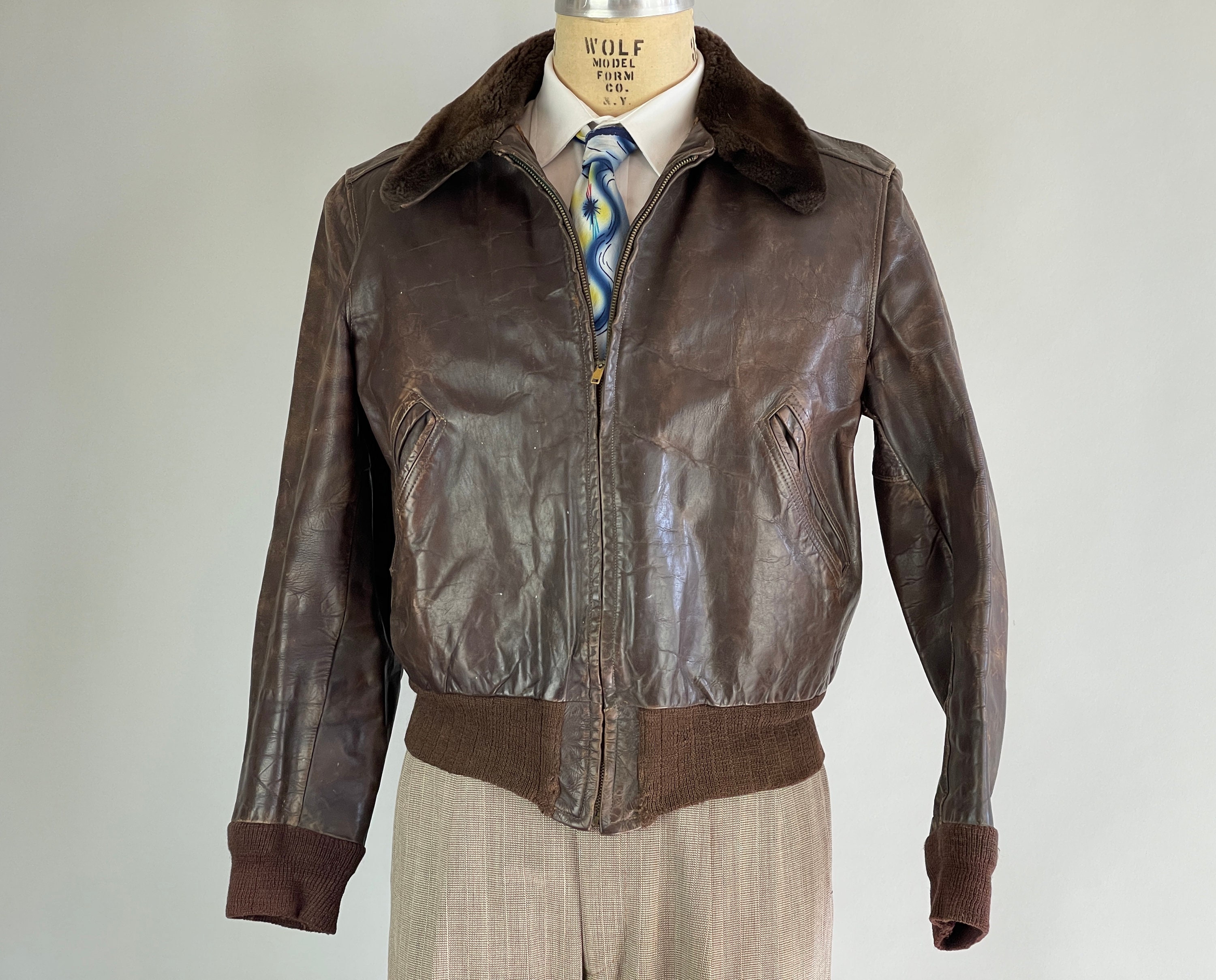The image features a vintage brown leather jacket, which appears to be from the 1950s or 60s, draped on a headless mannequin against a gray background. The jacket, which has noticeable crinkle marks suggesting its age, is only halfway zipped up. Underneath the jacket, the mannequin wears a white dress shirt paired with a tie that showcases a wavy pattern in blue, yellow, and white. Notably, the tie has blue stripes and yellow starbursts, accentuating its intricate design. The cuffs and bottom band of the jacket are made of suede, providing a contrast to the leather main body. The mannequin is also dressed in tan trousers with distinctive white lines. At the neck, a tan bandana with the inscription "Wolf Model Form Company" indicates the maker of the mannequin. The left sleeve of the jacket appears slimmer while the right one is notably thicker.